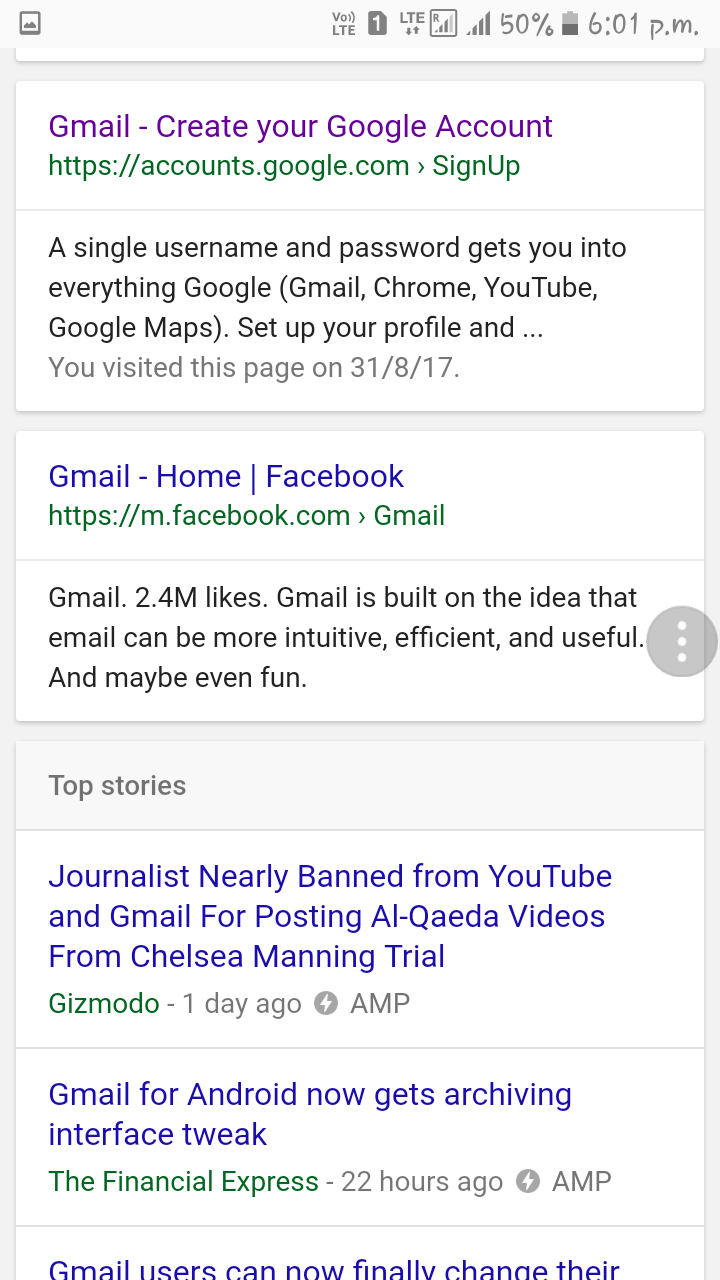The image depicts a phone screen with a Google search in progress. The background is light gray with a white upper section displaying a PNG icon, a V01 LTE icon, and several signal and battery status icons. From left to right, these include a single icon, another LTE icon, a box icon showing two signal bars, another icon with full four bars, and a battery icon indicating 50% charge at 6:01 PM.

Below the icons, the search bar contains the phrase "gmail - create your Google account" as the first link. The URL is https://accounts.google.com/signup, highlighted in green. The description states, "A single username and password gets you into everything Google: Gmail, Chrome, YouTube, Google Maps. Set up your profile in...". The note indicates that this page was last visited on 31.8.17.

The second link is labeled "gmail - home | Facebook" in blue, with the URL https://m.facebook.com/gmail in green. It reveals that Gmail has 2.4 million likes and describes Gmail as intuitive, efficient, and potentially fun. To the right, a gray circle with three dots appears.

Further down, in the "Top Stories" section, a gray area highlights a headline reading, "A journalist nearly banned from YouTube and Gmail for posting al-Qaeda videos from Chelsea Manning trial" in blue, attributed to Gizmodo in green, noted as "one day ago" in gray, accompanied by thunderbolt and AMP icons.

Another story reports, "Gmail for Android now gets archiving interface tweaked" in blue, from The Financial Express, 22 hours ago, with similar thunderbolt and AMP icons. A third headline starts with "Gmail users can now finally change their..." in blue, but the text is cut off, leaving the full content unread.

This detailed view of the phone screen provides a thorough context of the ongoing Google search and the information presented.